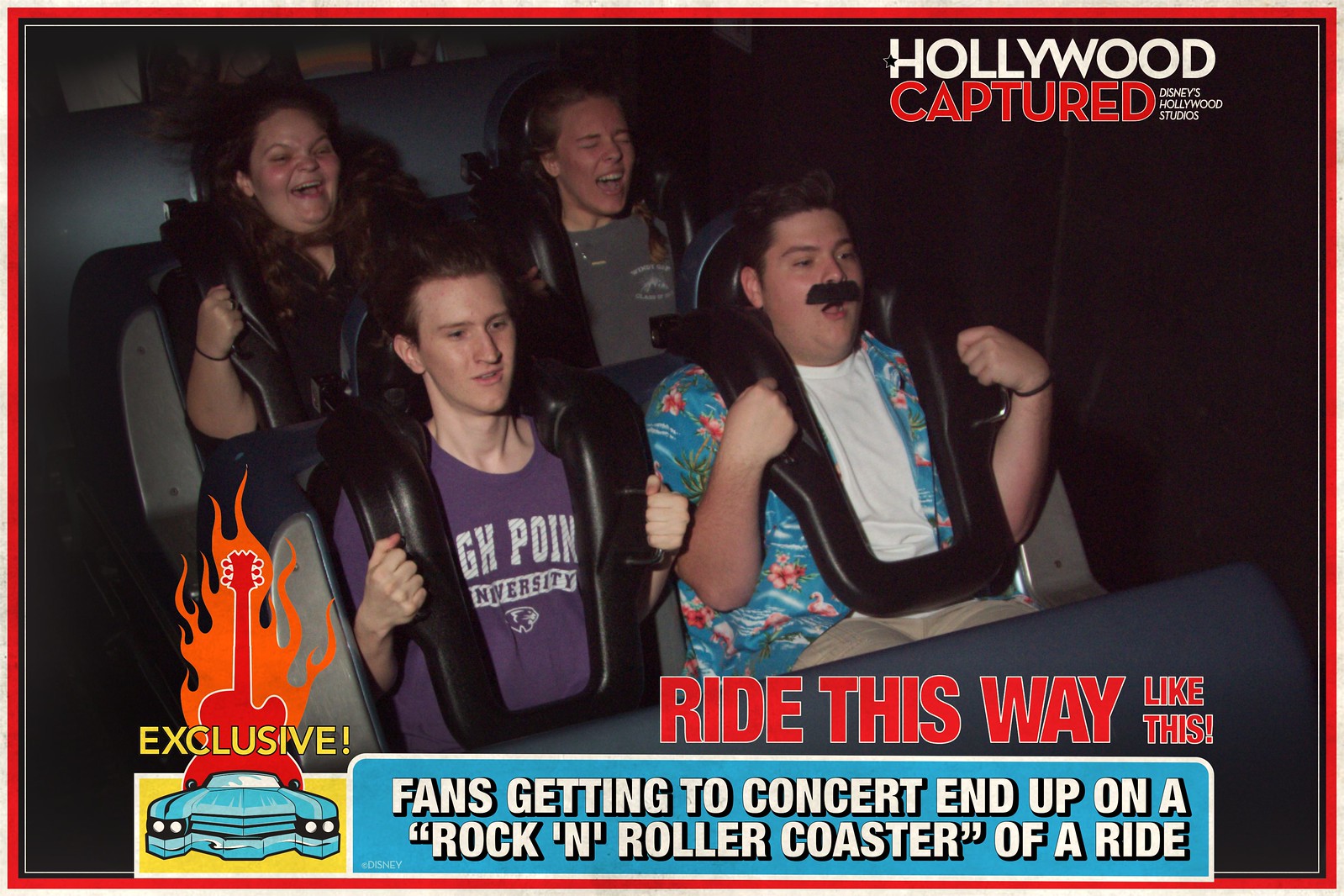This is a detailed night-time photograph set in an amusement park, specifically Disney's Hollywood Studios, capturing four people on a roller coaster ride. Central to the image are the individuals strapped into the ride with black leather harnesses, sitting on gray and blue padded seats. The photo composition places them in two rows: two are seated in the front and two in the back. The front right rider has a piece of black tape under his nose. The expressions reveal varying reactions - the back row occupants have their mouths wide open, with one keeping her eyes closed, while the front row riders have slightly open mouths, staring ahead.

Surrounding them, several colorful elements add vibrancy to the scene, with hues of black, white, gray, red, orange, yellow, light blue, purple, and green. Text elements provide context: "Hollywood Captured" and "Disney's Hollywood Studios" are prominently displayed at the top right. Below, on the left side over a blue car, red guitar, and orange flame, the word "exclusive" stands out. Towards the right, in red letters, the phrase "Ride This Way Like This" appears. Additionally, within a light blue box with white lettering, the text reads, "fans getting to concert end up on a rock and roller coaster of a ride." This photograph encapsulates the thrill and dynamic atmosphere typical of amusement park experiences, especially under the nighttime sky.